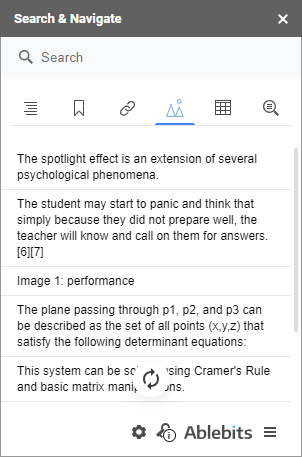In the image, the top portion features a screenshot with the words "Search and Navigate" displayed in white lettering on a grayish-brown background. Directly beneath this header is a search bar, accompanied by a magnifying glass icon and labeled with the word "Search."

Below the search bar, there are six distinct icons: 
1. An icon for alignment.
2. An icon for bookmarks.
3. An icon depicting a chain link.
4. An icon showing two small blue mountains with a circle above them.
5. An icon depicted as a grid.
6. An icon resembling a menu search icon.

Following this icon row, there is a section with dark gray text on a white background, reading: "The spotlight effect is an extension of several psychological phenomena."

In the subsequent section, the text suggests a scenario: "The student may start to panic and think that simply because they did not prepare well, the teacher will know and call on him for answers."

Further down, another section titled "Image One, Performance" appears. This is followed by a more detailed mathematical description: "The plane passing through P1, P2, and P3 can be described as the set of all points (X, Y, Z) that satisfy the following determinant equations." However, this content is interrupted by a white reload button featuring two arrows facing each other.

At the bottom of the image, there are three additional icons: a settings icon, an "Ablebits" icon, and a hamburger menu icon.